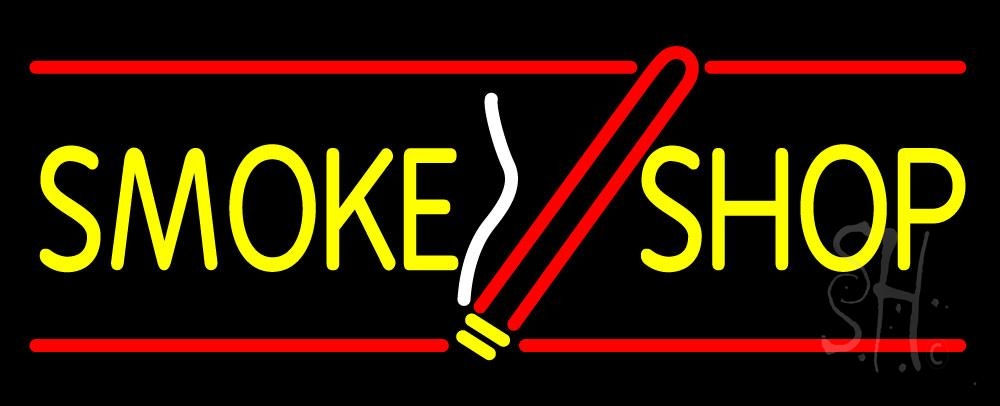The image features a long, black rectangular sign. Dominating the horizontal layout are bold, yellow capital letters that spell "SMOKE" and "SHOP," separated by a diagonally positioned, red, oval-shaped figure that resembles a cigarette. The "cigarette" bisects both the top and bottom edges, with the base defined by a red, upside-down U shape along with an additional white zigzag to represent smoke. Red horizontal lines stretch across the top and bottom edges of the sign. In the bottom right corner, a subtle, light gray logo appears, featuring two stacked 'S' shapes with an 'H' beneath them, which is etched lightly and partially obscured by the bold background. The entire design emits a bright, illuminated effect, typical of a light-up store sign.